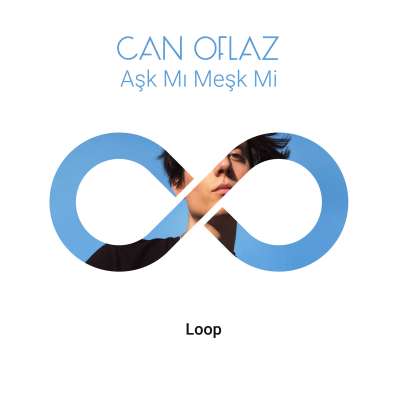This digital image features a central infinity symbol containing a man's face. Above the infinity symbol, in the top middle of the image, is blue text that reads "can of less ask me mask me." Below the infinity symbol, in the bottom middle of the image, black text reads "blue" or "loop." The background of the image is white, with additional colors including light blue, black, tan, and pink. This appears to be a logo, possibly for a company, set against a background suggesting that it could be used on a business card or a company website.